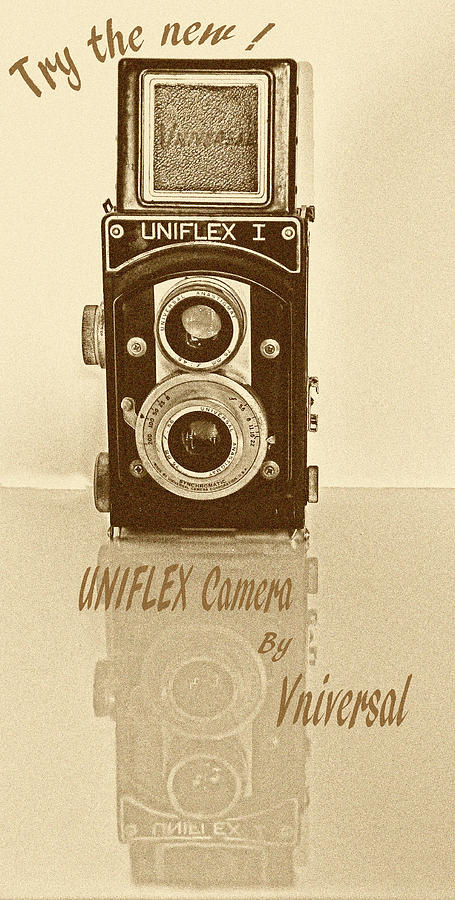This advertisement showcases the Uniflex 1 camera by Universal. Dominating the center of the image, the sleek, black and white camera is portrayed with a polished reflective surface beneath it, giving the effect of being placed on water. The camera features two main lenses, various knobs for adjusting settings and capturing images under different lighting conditions, and a small screen. The background is a light tan yellow stone color, gradiently darkening towards the edges. The tagline "Try the new!" is prominently displayed at the top of the image, while the bottom of the advertisement reads "Uniflex camera by Universal" in a darker khaki-colored print. Attention to detail and precision in its vintage-inspired design suggest both a nod to nostalgic appeal and modern functionality.